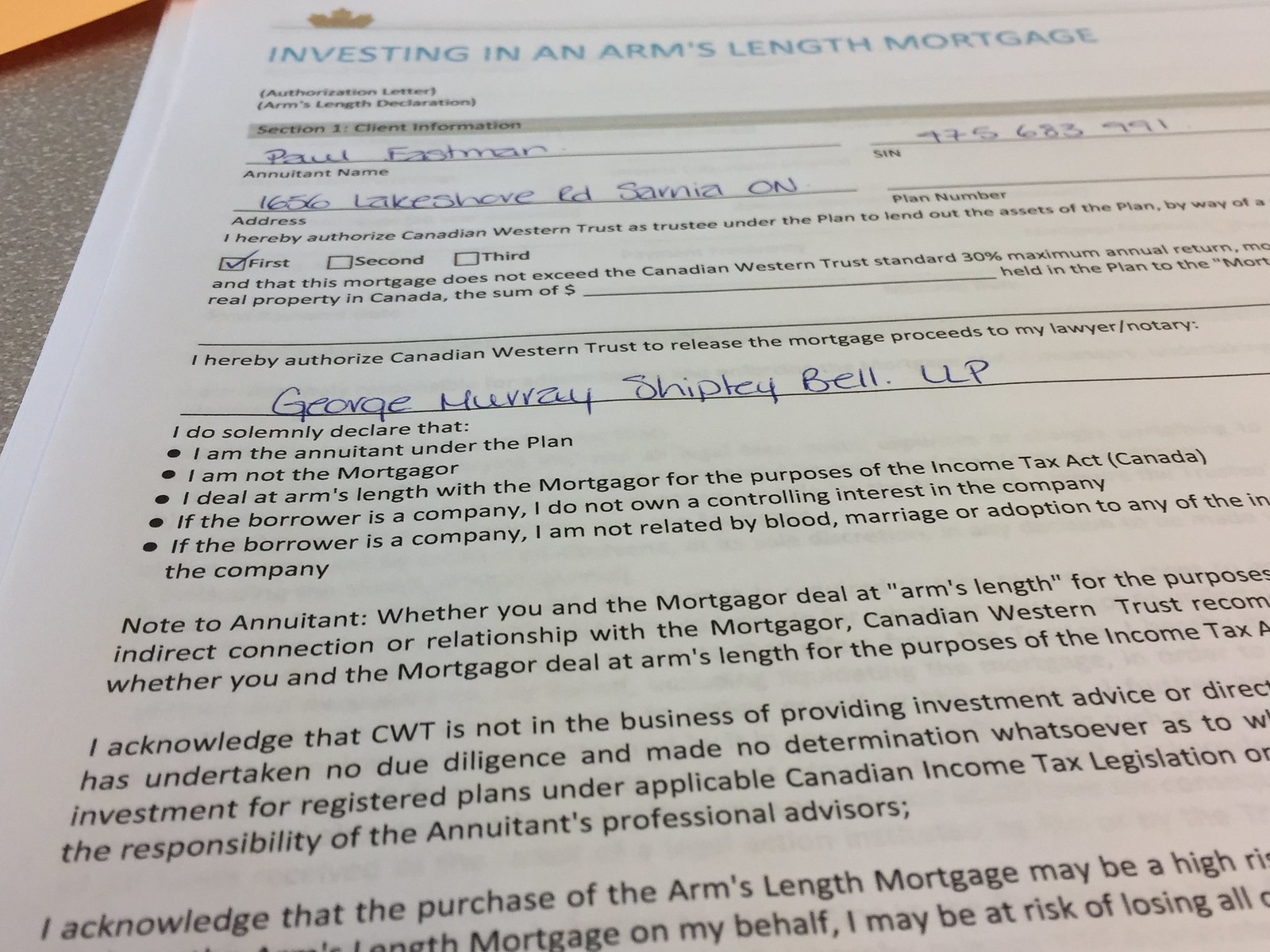The image is a detailed photograph of a filled-out form titled "Investing in an Arm's-Length Mortgage," which is printed in light blue at the top. The form is placed on a table alongside other papers. The form appears to be an authorization letter and arm's-length declaration with various sections for a client to fill out. 

The first section contains client information, filled in blue pen. It includes the name Paul Eastman and a Social Insurance Number (SIN) 475-683-991. Below that, the address is provided as 1656 Lakeshore Road, Sarnia, ON. There is a black-typed section where Paul authorizes Canadian Western Trust as trustee to lend out assets from the plan, with three checkboxes where the first option is ticked. 

Another part of the form states, "I hereby authorize Canadian Western Trust to release the mortgage proceeds to my lawyer/notary," with the name George Murray Shipley LLP written in blue pen. The form has a declaration section stating the signer is not the mortgager, deals at arm’s length with the mortgager, and has no substantial interest in the borrower company. The right-side text of the form is slightly cropped out, missing some details.